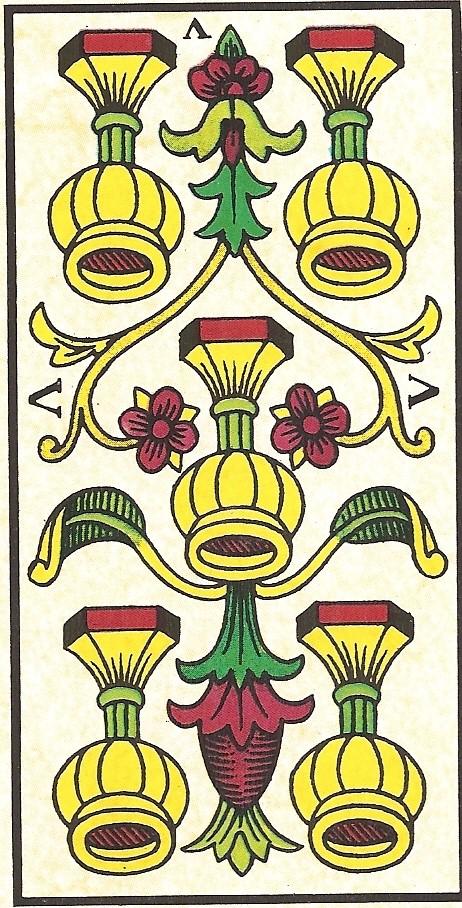This graphical image features a vertically stretched, thin, narrow design that prominently includes text and depicted elements which suggest that the entire composition might be viewed upside down. Central to the imagery are five identical goblet-like objects, displayed in bright yellow with green stems and red bases. These elegant goblets, which resemble ornate lamp bases, are arranged symmetrically. Two goblets are positioned at the top of the image, one in the center, and two more near the bottom.

The background is predominantly white, adorned with striking decorative elements that further enhance the symmetrical appearance. Flourishing across the backdrop are intricate, flowery vines with yellow stems and scattered green leaves. These vines feature red and yellow flowers, adding vibrant splashes of color. Among the floral arrangement, one vine stands out as it grows towards the top of the image from the central goblet, culminating in an unbloomed flower bud with yellow peaks, adding a touch of anticipation and beauty.

The overall composition suggests a blend of artistic creativity and symmetry, evocative of ornamental styles perhaps reminiscent of tarot card designs, although the exact nature remains open to interpretation.